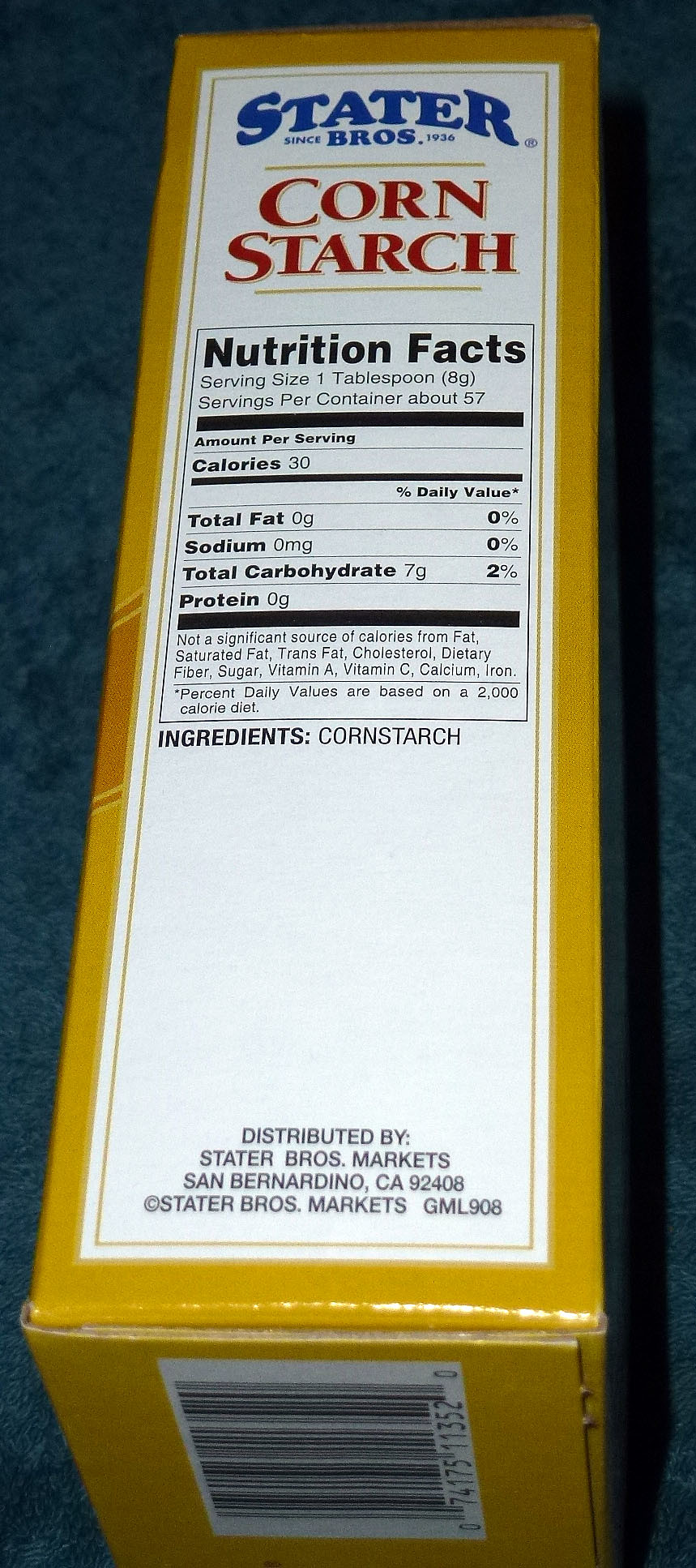The image features a focus on the side panel of a yellow box with a white label. The top section of this panel prominently displays the word "Cornstarch" in bold red letters, clearly identifying the contents of the box. The brand, Stater Brothers, is written in blue letters at the very top of the white panel, signaling the company's ownership. Directly below the word "Cornstarch," the label reads "Nutrition Facts" in black letters, though the details such as serving size and servings per container are slightly out of focus. At the bottom of the side panel, we see additional information stating the product is distributed by Stater Brothers Markets, located in San Bernardino, California, 92406, followed by the text Stater Brothers Markets, GM, L908. The barcode is also visible at the bottom of the box, adding to the comprehensive labeling on the side panel.